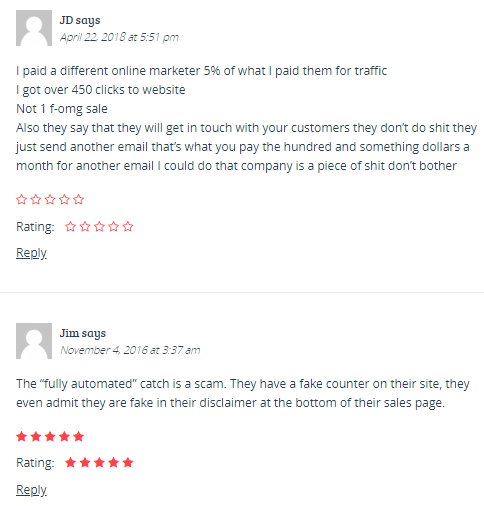In this image, there is an article or piece of text by "JDay Sales" prominently displayed. The first entry is dated April 22, 2018, at 5:51 PM, presumably from a user who expresses deep dissatisfaction with a marketing service. The user states that they paid another marketer only 5% of what they paid JDay Sales for traffic, resulting in over 450 clicks to their website but not a single sale. They criticize the company's customer service, claiming that instead of getting in touch with customers, JDay Sales merely sends another generic email. The user describes the company in derogatory terms and advises others not to engage with them, pointing out the lack of ratings.

There is a reply button below this entry, and a second entry from the same user named Jim, dated November 4, 2016, at 3:37 AM. In this post, Jim labels the "fully automated catch" from the company as a scam and accuses them of using a fake counter on their site, which they apparently admit to in a disclaimer at the bottom of their sales page. Despite these issues, this post is oddly rated 5 stars, with a 5-star rating visible next to it. Another reply button is featured beneath this second entry. The text on the image is black, set against a white background, making the details clear and legible.